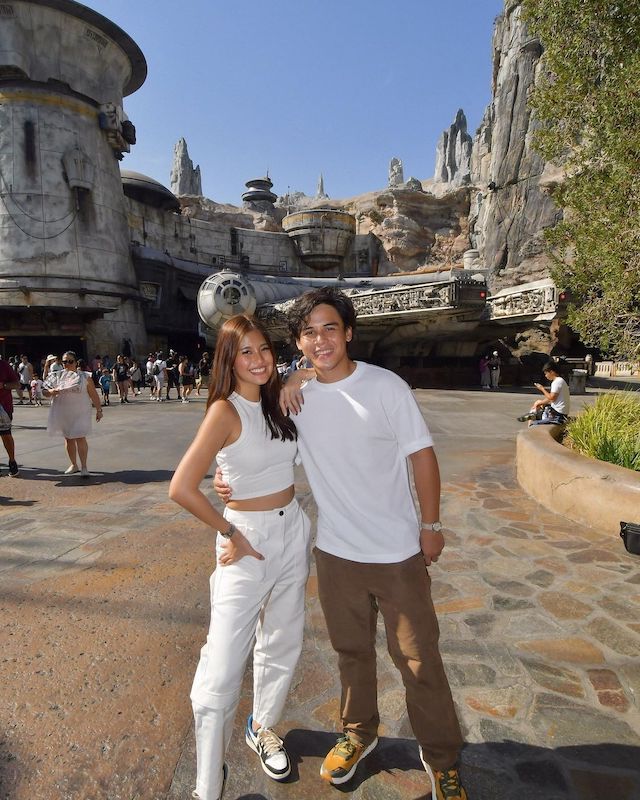In this detailed photo taken at what appears to be Disneyland in the Star Wars-themed area, two people, likely in their mid-twenties stand in the foreground on a paved, concrete street patterned with brown and black prints. The woman on the left, with long brunette hair, is wearing a white tank top and white jeans with a midriff. She completes her outfit with kids-like shoes and standing confidently with her right hand on her hip, while her left arm gently rests over the shoulder of the young man beside her. The man, wearing a white t-shirt, brown khaki pants, and yellowish trainers with white trims, has his right arm wrapped around the woman's waist. Behind them, a medieval, city-like structure built into rugged gray-white rocks rises dramatically, featuring turret-topped buildings that resemble concrete temples or cathedrals. The iconic Millennium Falcon ride, set amid a theme inspired by the Star Wars universe, is partially visible in the backdrop along with several tall, city-like rock structures. Other park-goers mingle around in the bustling background, adding to the lively atmosphere of this captivating scene.